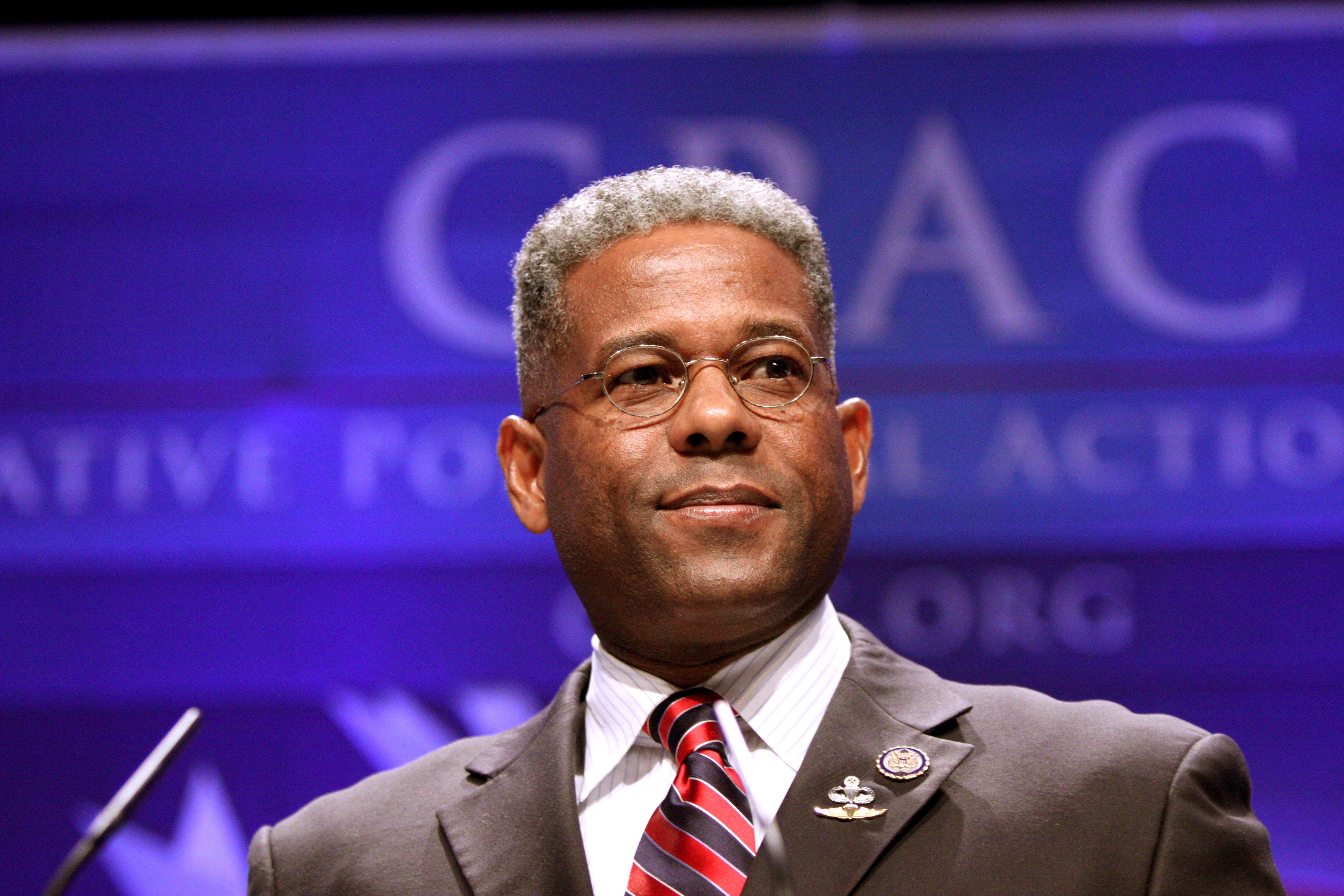The image is a photograph taken at a conference, featuring a black man with short, predominantly grey hair, who appears to be on a stage. He stands in front of a mounted thin microphone, which is positioned to his left, and gazes off to the right with a slight smile on his face. He wears thin-framed, silver-rimmed round glasses, and sports a dark grey suit jacket adorned with two lapel pins. His white buttoned-up shirt is complemented by a red and dark blue striped tie. The background behind him is predominantly blue with a large purple sign or projector screen displaying the text "CPAC" and a partially visible .org website. The sign appears out of focus with its top line in bold white font, contributing to the professional atmosphere of the conference setting.